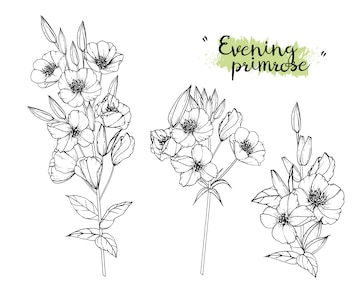The image features three sketched drawings of Evening Primrose flowers, labeled at the top with the text "Evening Primrose" in bold black cursive, accented with a wavy line of sage green underneath. The text is encased in quotation marks. The flowers, depicted in black and white pencil sketch, are arranged in three distinct bundles. 

The bundle on the far left is the largest and most detailed, with a tall, leafy stem supporting multiple layers of blooms, each flower showcasing five petals. The middle bundle, of medium height, includes a slender stem with several visible blossoms and a few buds yet to open. The smallest bundle on the right resembles a boutonniere, featuring two prominent flowers, accompanied by additional buds and leaves at the base, with the stem less visible. The background of the sketched flowers remains monochromatic, contrasting with the subtle green hue beneath the floral text.